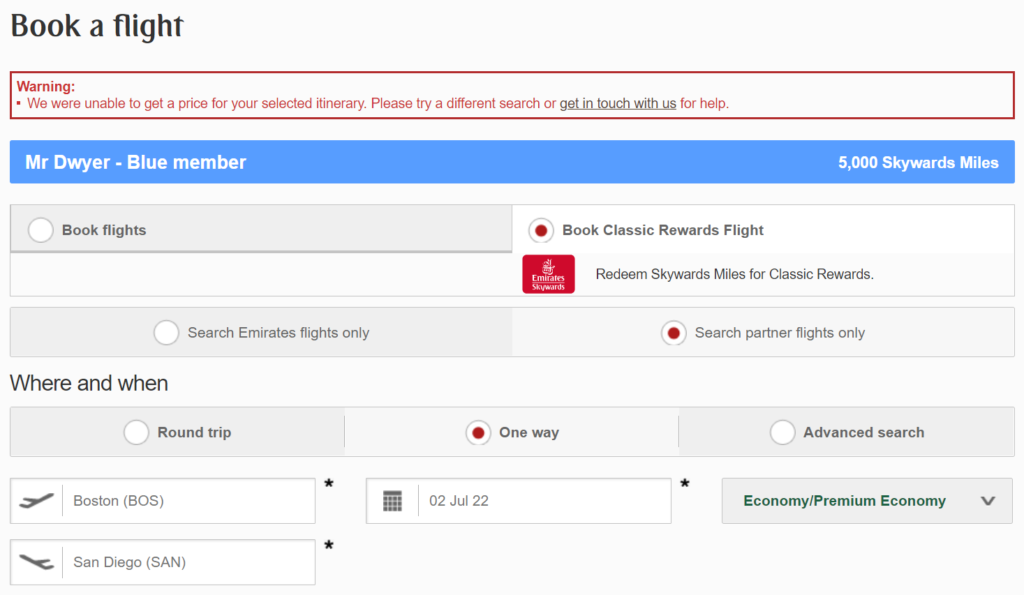**Detailed Caption:**

A screenshot of a webpage where an individual is attempting to book a flight. At the top, the page headline reads "Book a Flight." Directly below, there is a prominent red box displaying a warning message: "We were unable to get a price for your selected itinerary. Please try a different search or get in touch with us for help." The phrase "get in touch with us" is underlined and in black text, standing out from the rest of the red text.

Further down, there is a blue box containing white text indicating the user's name, "Mr. Dwyer," followed by the designation "Blue Member." To the right of this box, it states that Mr. Dwyer has "5,000 Skywards Miles."

Below this section, there are options to "Book Flights" or "Book Classic Rewards Flight," with the latter being highlighted. An Emirates Skywards logo is also visible, emphasizing the option to redeem Skywards Miles for Classic Rewards. Additional selection options include "Search Partner Flights Only" or "Search Emirates Flights Only," with the "Search Partner Flights Only" option chosen.

In the area labeled "Where and When," various travel options such as "Roundtrip," "One-Way," and "Advanced Search" are available. The user has selected "One-Way." They have chosen "Boston" as the departure city and "San Diego" as the arrival city, with the departure date set for July 2, 2022. The travel class selected is "Economy/Premium Economy," indicated by green text and accompanied by a drop-down button.